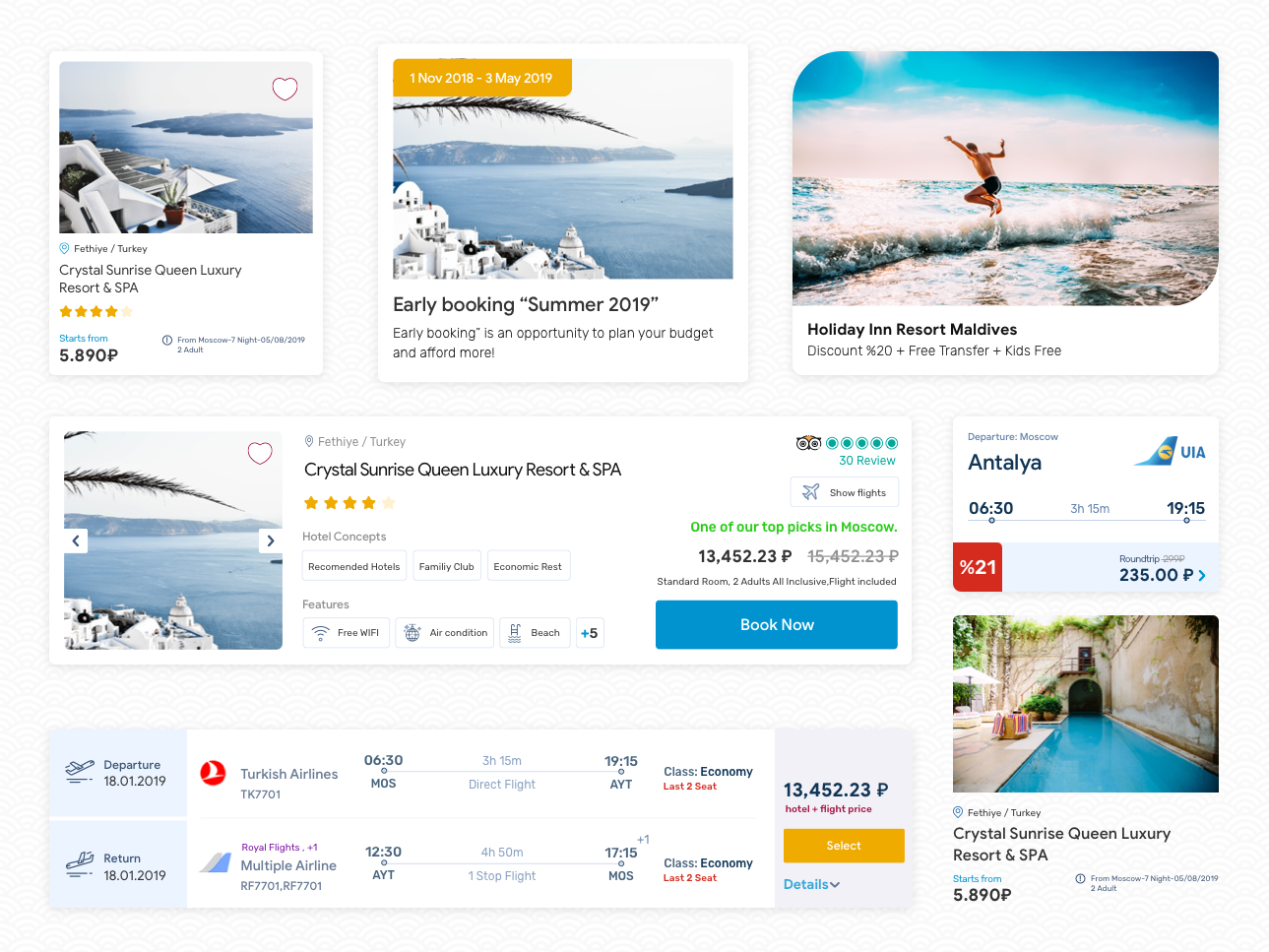The image features a white background with multiple sections and images showcasing holiday packages and flights. 

**Top Left Section:**
- A photo of a serene spa area with a body of water and lounge chairs.
- Text above the image reads: "Crystal Sunrise Queen Luxury Resort and Spa."
- Rating: 4 out of 5 stars.
- Price: Starts from $5,890 (currency not specified).

**Middle Section:**
- Promotion image with text: "Early Booking, Summer 2019. Early Booking is an opportunity to plan your budget and afford more."
- Photo of white buildings along a waterfront.

**Next Image:**
- Details for "Holiday Inn Resort, Maldives" featuring:
  - Discount: 20% off
  - Free transfer
  - Kids stay free

**Below Initial Image:**
- "Crystal Sunrise Queen Luxury Resort and Spa" detailed listing:
  - Rating: 4 stars 
  - 30 reviews
  - Noted as one of the top picks in Moscow
  - Price: $13,452.23 (currency not specified)
  - Standard room for two adults, all-inclusive, flights included
  - A blue "Book Now" button

**Right Section:**
- Flight details: 
  - Departure from Moscow to Antalya via UIA 
  - Time: 6:30 to 19:15
  - Additional 20% off and price note: 235P (currency not specified)

**Below Flight Details:**
- Additional departure listing for Turkish Airlines:
  - Time: 6:30 to 19:15

- Return flight details with multiple airlines:
  - Time: 12:30 to 17:15
  - Price: $13,452.23 (currency not specified)
  - Option to select flight package

The overall layout is designed to offer travel packages and flight details prominently, with clear pricing and special offers indicated.